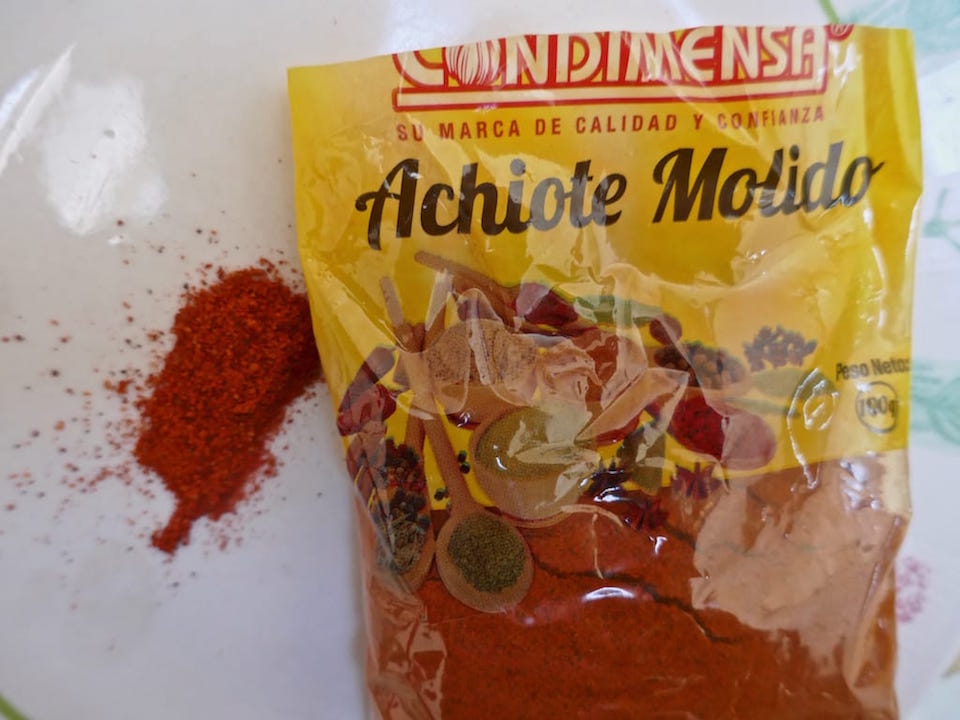This image showcases a vibrant, shiny plastic bag of chili powder, prominently placed on a white surface. The bag, heavily filled with this dark red seasoning, has been opened, with some of the powder spilled out and forming a small pile on the left side of the image. The packaging features the brand name "Condimensa" at the top, albeit with some letters cut off due to the top part being snipped off. Below this, it proudly displays the phrase "Su Marca de Calidad y Confianza," indicating quality and trust in Spanish. The bag also displays various culinary illustrations such as two spoons, bowls filled with seasonings, and a section depicting artichoke, tea, and molybdenum patterns, all against a yellow backdrop on the right side. On the middle right side, it notes "Pesto Lettuce" with a circle labeling "190 grams" beneath it. The bag is labeled "achiote molido," suggesting it's a type of ground pepper, although it might not be clear in English.